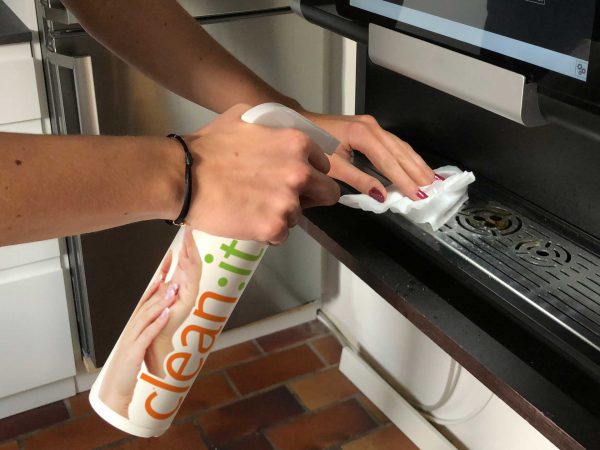In the photograph, a pair of hands are meticulously cleaning a kitchen appliance. The hands, which appear to belong to a woman, feature red painted fingernails and are adorned with a black bracelet on the right wrist. The right hand grips a tall white spray bottle displaying an orange and green label with the text "CLEAN IT" and an image of two hands rubbing together. This bottle is being used to spray a cleaner onto a stainless steel beverage dispenser grate. The woman's left hand is pressing a white cleaning cloth against the grate, which is speckled with white spots from the cleaner. The appliance being cleaned is situated in a kitchen that also features a stainless steel refrigerator in the background. The scene is set against a backdrop of brick flooring, white cabinets, and other stainless steel kitchen appliances, indicating a modern, well-maintained home kitchen.